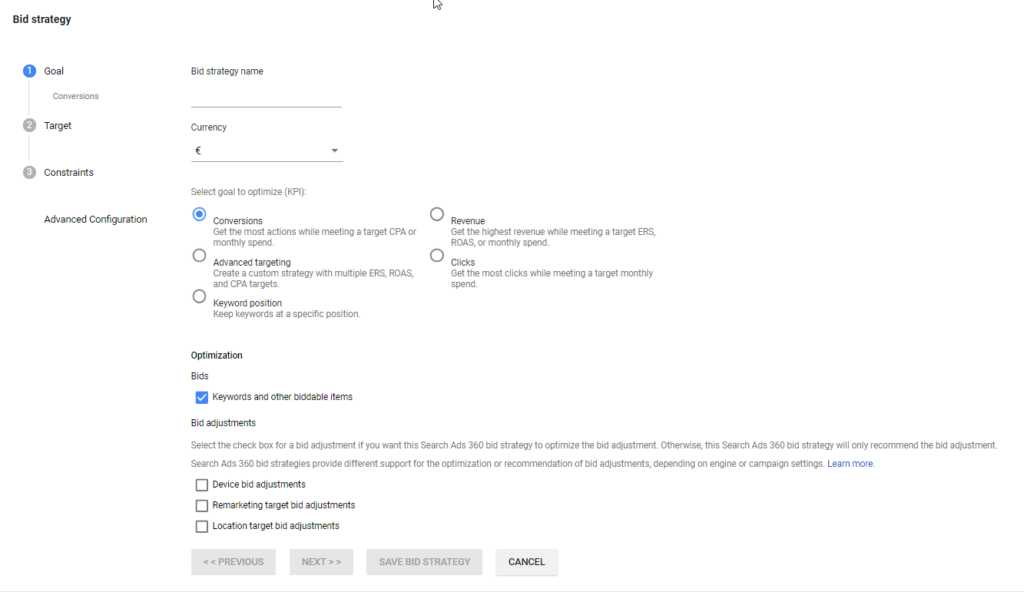The image is a screenshot with a pure white background featuring various text elements, most of which are blurry and rendered in light gray. However, some darker and clearer words stand out. 

In the top left corner, bold black letters spell out "BID STRATEGY." Below this heading, three circles in a vertical sequence denote steps or categories: 
1. A blue circle labeled "GOAL."
2. A gray circle labeled "TARGET."
3. A gray circle labeled "CONSTRAINTS."
Beneath these, a standalone phrase "ADVANCED CONFIGURATION" appears.

Centrally positioned in the image, the text reads "BID STRATEGY GAME," followed by a gray horizontal line. Below this line, the word "CURRENCY" also sits above another gray horizontal line. There is a drop-down box indicated by a gray triangle pointing downward, though the specific currency symbol within this box is indiscernible.

Further down, some light gray text possibly reads "SELECT GOAL TO OPTIMIZE" with "KPI" in brackets. A white circle outlined and centered in blue contains the word "CONVERSIONS" in black. Below this, a series of topics are listed:
- "ADVANCED TARGETING" next to an unselected circle.
- "KEYWORD POSITION" next to another unselected circle.
- A circle next to the word "REVENUE," though accompanying light gray text is unclear.
- The word "CLICKS" in black, followed by more light gray text.

Lower in the image, bold black text states "OPTIMIZATION" and underneath it, "BIDS." A blue square with a white checkmark is adjacent to the phrase "KEYWORDS AND OTHER BIDDABLE ITEMS." Below this phrase, the words "BID ADJUSTMENTS" appear, followed by two lines of indistinct light gray text.

Three vertically stacked white squares bordered in black are next to these lines, each corresponding to specific bid adjustments categories:
1. "DEVICE BID ADJUSTMENTS."
2. "REMARKETING TARGET BID ADJUSTMENTS."
3. "LOCATION TARGET BID ADJUSTMENTS."
All boxes remain unticked.

Towards the bottom of the image, gray boxes contain navigation and action buttons labeled "PREVIOUS," "NEXT," "SAVE BID STRATEGY," and "CANCEL," with the "CANCEL" button in bold black letters. The rest of the text remains too unclear to decipher further.